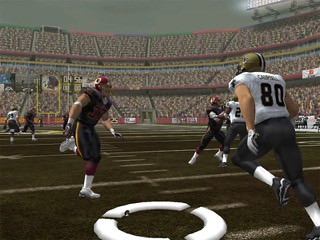A screenshot captures a moment from a football video game, seemingly played on either a TV or a PC, showcasing an intense stadium atmosphere filled with virtual spectators. The action centers around a kickoff, where the team resembling the New Orleans Saints, clad in their traditional black and white uniforms, has just kicked the ball high into the air. The opposing team, dressed in the maroon, gold, and black colors reminiscent of the Washington Football Team (formerly known as the Redskins), is poised to catch and return the kickoff. The vibrant stadium, packed with cheering fans, adds to the electrifying atmosphere of this simulated football showdown.